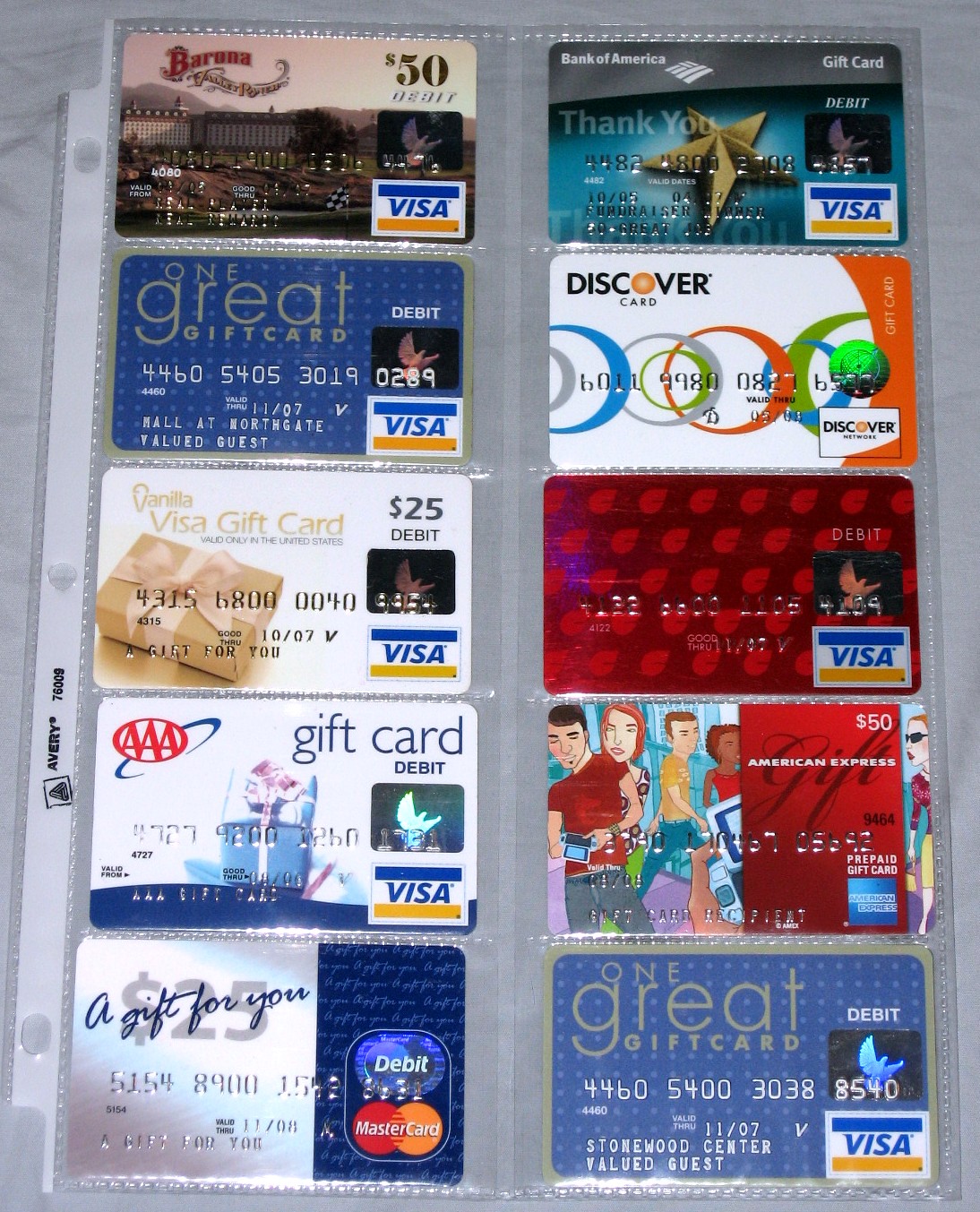This photograph captures a collection of 10 credit and debit cards, primarily composed of Visa gift cards, among them also a MasterCard, an American Express card, and a Discover card. Each card features a unique design, ranging from a blue present with a AAA logo, a red card with decorative splotches, to an animated group of young people shopping and a golden star. The cards are neatly arranged within a plastic protective sheet, displayed much like family photographs, lying flat on a marble white table. The cards vary in value, predominantly marked at $25 and $50, with one notable Visa card displaying an image of a building. The overall composition and varied designs suggest they come from different banks and organizations.